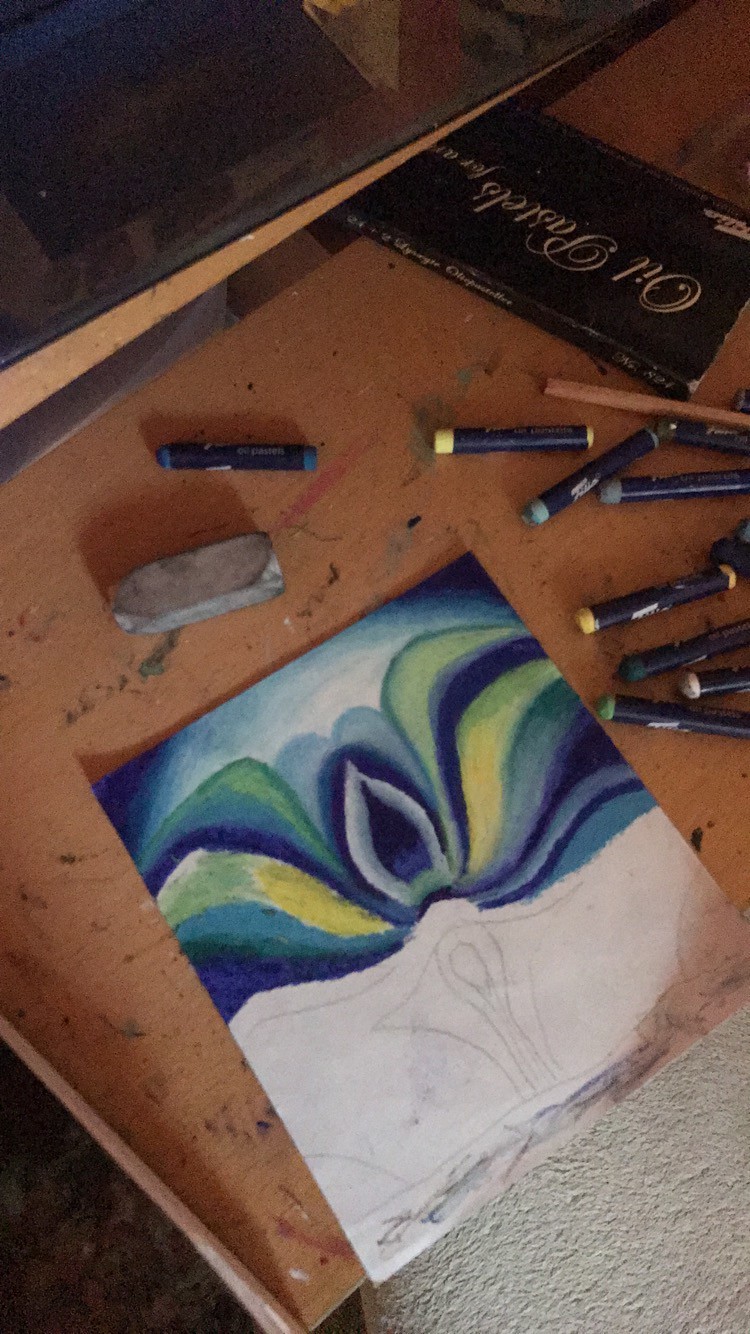This color photograph showcases an artist's well-used wooden work table, bearing numerous marks from oil pastels and colored pencils. The focal point is a half-finished oil pastel drawing on a square piece of paper. The artwork depicts a blue flower with its lower half still in pencil outlines, awaiting color. The flower's upper half is richly textured with blended streaks of blue, green, yellow, and white, converging into an oval shape that evokes the style of Georgia O'Keeffe's floral depictions. Scattered around the drawing are oil pastel crayons, still wrapped in their black packaging. A large, square eraser is positioned directly above the art piece, and an overturned black box labeled "Oil Pastels for Art" lies nearby. The image is notable for its grainy texture and cinematic aspect ratio, indicating it was taken with a phone camera.